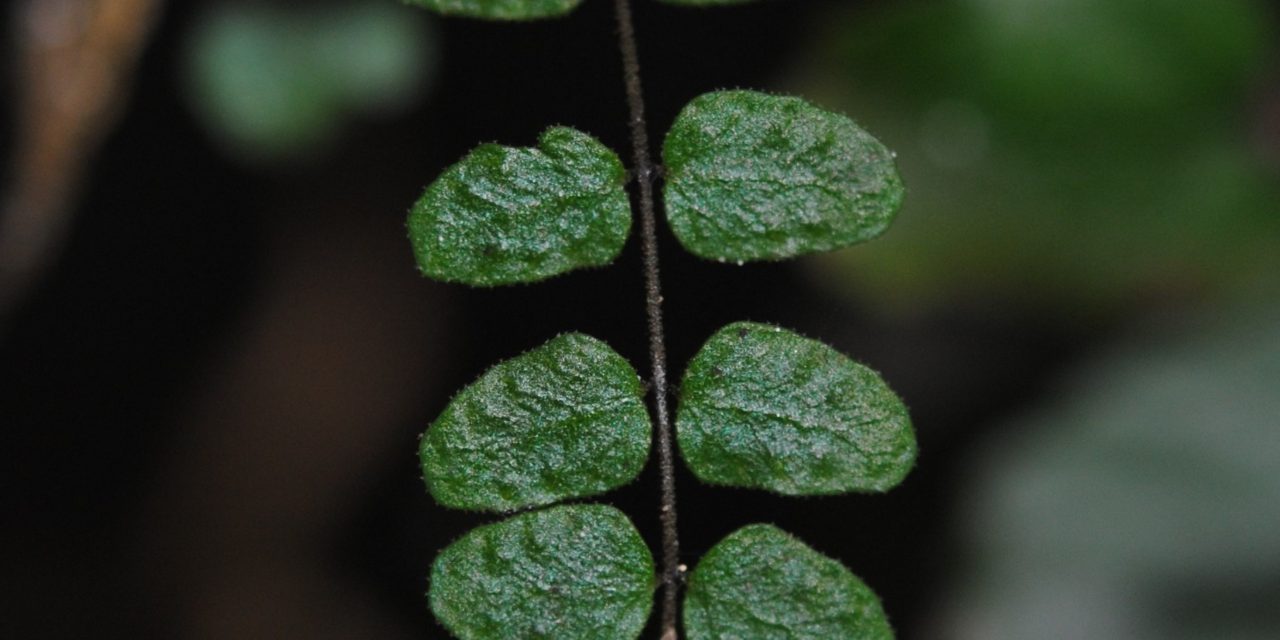This high-definition photograph presents a close-up view of a slim, blackish-brown branch running vertically through the center of the frame, intersecting the middle of the image almost symmetrically. The composition features three pairs of vibrant green leaves, making up a total of six leaves, each pair emerging oppositely from similar points along the branch. The dimensions of the photograph extend wider than taller, akin to a high-definition TV screen. Each pair of leaves is positioned so that two pairs appear near the bottom, closely grouped, while another pair is spaced further apart towards the top. The leaves at the bottom, which are slightly shinier and very green, are partially visible, with some edge parts cut off by the bottom frame. The background, though blurred, contributes a soft mix of black, brown, green, and white hues, enhancing the focus on the branch and its verdant foliage.